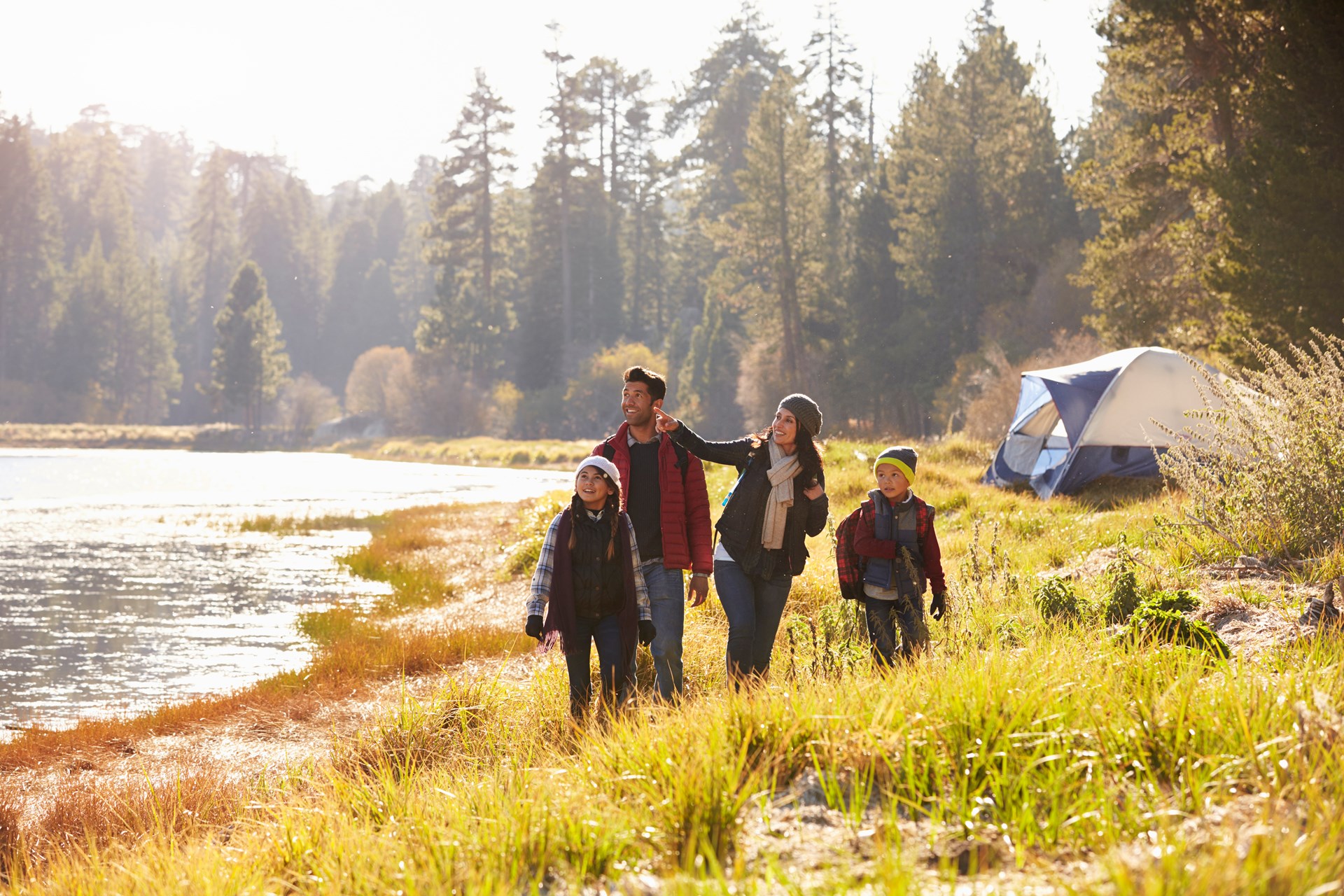This vibrant color photograph captures a family of four—the father, mother, young boy, and preteen girl—enjoying a day in nature by the serene lakeshore. The backdrop features a forest of tall, towering spruce trees and lush, shorter willow-like trees, adding depth and beauty to the scene. The bright sun illuminates the sky, water, and ground, casting a radiant glow across the entire image. The family stands amidst the high grasses along the lake's edge, with a blue and white tent set up to the right. All members are warmly dressed, indicating it's likely fall; they wear jackets, jeans, and knit hats. The mother, wearing a green hat, a black jacket, and blue jeans, points upwards and to the left, drawing everyone's gaze in that direction. The father, in a red puffy jacket and blue jeans, stands beside her, while the young boy, dressed in a flannel shirt with a blue vest and jeans, and the preteen girl, wearing a flannel blue shirt, blue jeans, and a white hat, look on in anticipation. The bright sunlight reflects off the water to the left, obscuring its color but enhancing the overall brightness and beauty of this idyllic family moment.